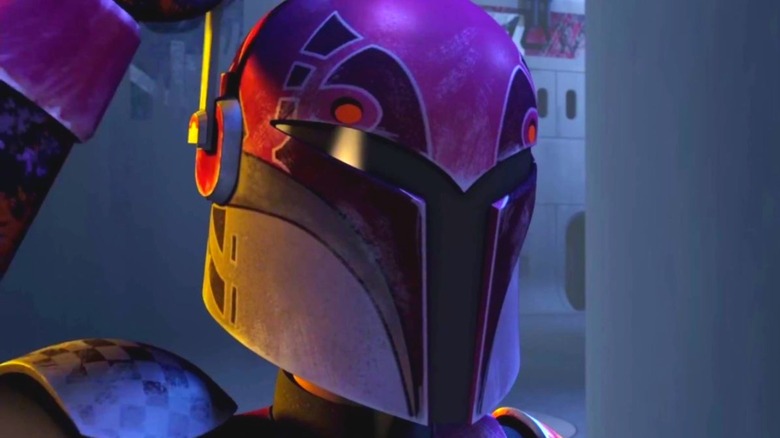In this detailed horizontally aligned rectangular animated image, we see a close-up of a helmeted figure prominently displayed at the center. The helmet, which extends past the chin, is adorned with a purple on the top, transitioning to lighter purple and black sections. The forehead area is decorated with square and curved shapes with purple outlines around black-shaded zones resembling eyebrows. The distinct black Y-shaped section on the front runs from above the eye area down to the nose, flanked by additional black sections. Notably, the helmet features red detailing at the ear on the left side, complemented by a silver antenna extending upward.

The figure's right shoulder is partially visible, showcasing checkered light blue and dark blue armor, while the left shoulder pad appears in a checkered pattern of purple and black. The arm on the left seems to be raised, with a bent elbow and a purple metallic cuff on the wrist visible towards the upper right corner. The background primarily consists of dark gray stone walls, with a hint of purple accents identical to the helmet's hue. A segment resembling a cement wall is also discernible on the right side of the image, providing a stark, industrial contrast to the vibrant colors of the armor.